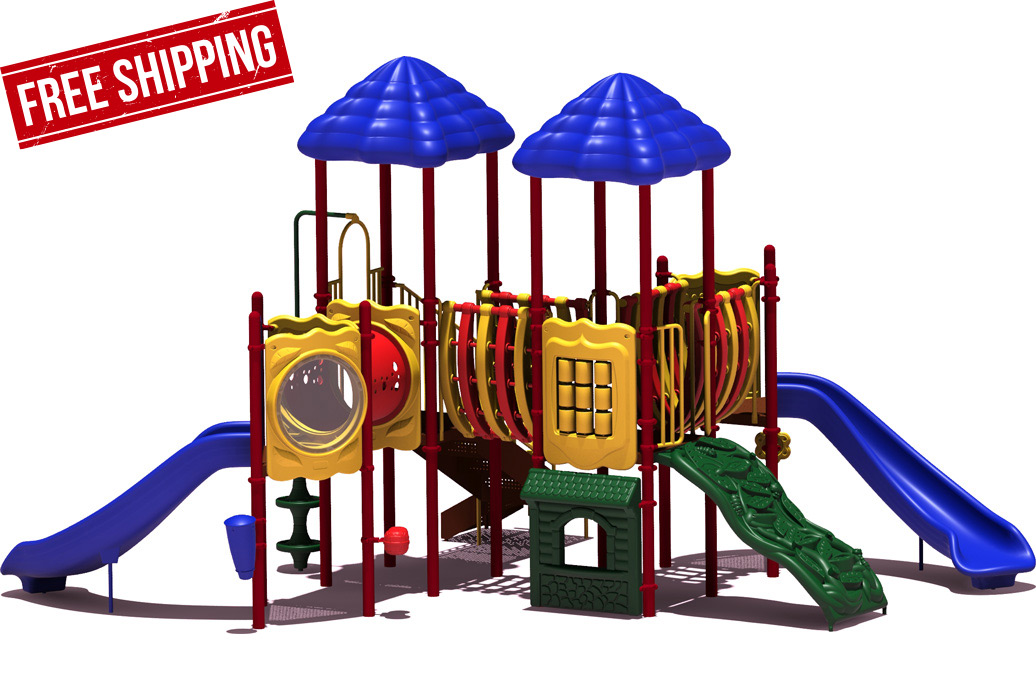The image depicts a children's plastic playground set against a plain white computer screen background, making it difficult to gauge its actual size. The playground, potentially suitable for a backyard, school, or park, features a traditional design with vibrant primary colors. It includes two blue slides positioned on either side, two blue pyramid-shaped canopies, and a pair of half domes supported by poles at the front. The structure also boasts multiple ways to ascend: stairs, a green climbing ladder, and other climbing components. In addition to these, there are nine rotating cylinders and tubular elements for climbing or walking through. Most of the playground elements are colored blue, red, yellow, and green. The image also prominently displays a red banner in the upper left corner that advertises "free shipping."